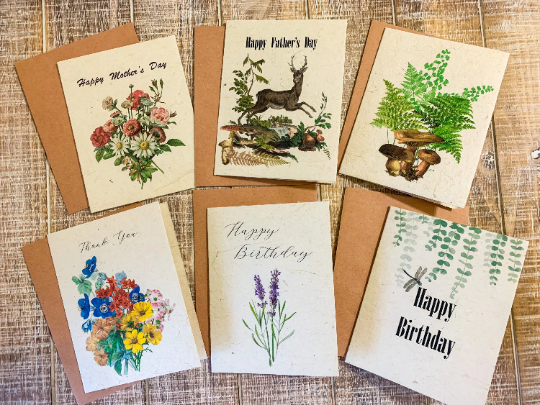This image showcases six greeting cards arranged on a medium brown wooden table, each accompanied by a light brown envelope. 

- The top left card reads "Happy Mother's Day" and features a vibrant array of white flowers with yellow centers, red flowers, and a pink flower, all set against abundant green foliage.
- The upper middle card says "Happy Father's Day" and depicts a dark brown deer with antlers amidst branches, leaves, and faint floral details, with some twigs and perhaps tree bark below.
- The top right card displays a botanical illustration of greenery and three large mushrooms, with no text.
- The bottom left card is a thank you card adorned with a mix of yellow, red, peach, blue, and turquoise flowers interspersed with green leaves.
- The lower middle card says "Happy Birthday," showcasing what appears to be lily of the valley or possibly purple violets accompanied by green leaves.
- The bottom right card also says "Happy Birthday" in black letters, featuring a small gray dragonfly above the "H" and green leaves extending from the top border to the card's middle.

All the cards share a white background and are paired with light brown envelopes.